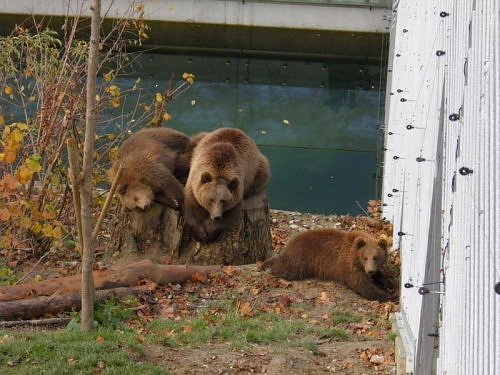This photograph captures a zoo enclosure featuring three light-colored brown bears, tinged with a reddish-orange hue. The scene unfolds behind a distinct heavy metal gating system adorned with black eye hooks, indicative of electrical or cable support structures. Behind the bears, a concrete and possibly water-filled pit with a bluish hue suggests a cooling area for the animals, especially useful during hot summers. 

Central to the image, two bears rest atop a sizable tree stump. One, possibly the mother, is dozing with its front legs draped over the stump's edge, facing the camera. Adjacent to it lies another bear, potentially an adolescent, sound asleep on its side with its head tucked under its front arms. To their right, a cub lies on its belly, appearing awake yet groggy, staring inquisitively at the viewer. The enclosure also houses a sparse, barren tree and scattered logs, amidst patches of grass and dirt, painting a picture of either late fall or early spring. The white concrete wall on the right provides a stark backdrop to this tranquil setting.